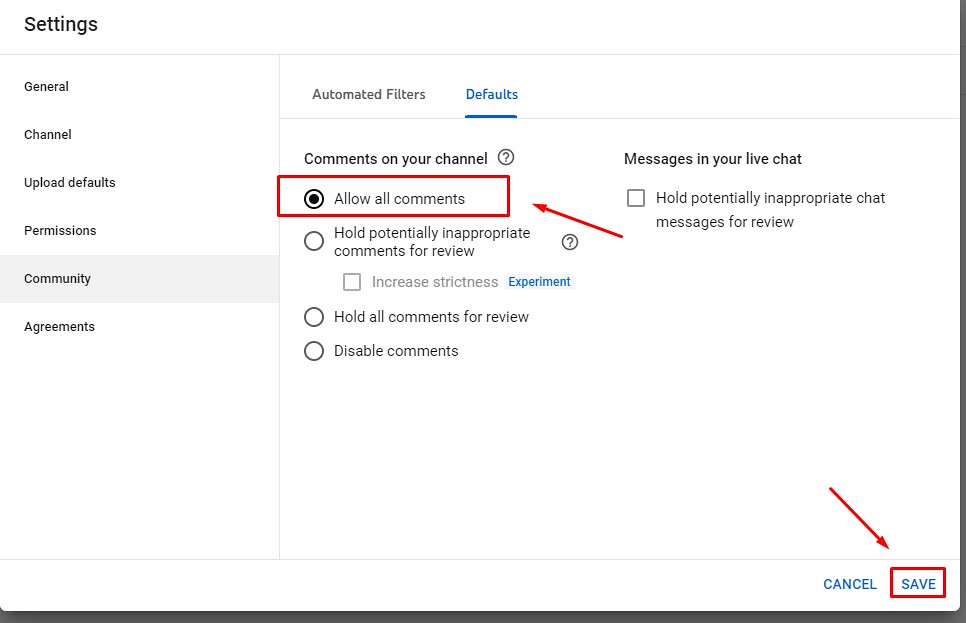This image appears to be a screenshot from a YouTube settings tutorial. The background is entirely white with black text. In the top-left corner, "Settings" is prominently displayed, and beneath it is a horizontal gray line that spans across the page. To the left, there is a vertical list of clickable headings: 

- General
- Channel
- Upload Defaults
- Permissions
- Community (highlighted with a gray box around it)
- Agreements 

On the right half of the page, there are two main headings: "Automated Filters" and "Defaults." The "Defaults" heading is selected, appearing in a bright blue color and underlined, while "Automated Filters" is in dark gray.

Under the "Defaults" section, there is an option labeled "Comments on your channel," accompanied by a question mark inside a circle, presumably to get more information. The selected option is "Allow all comments," indicated by a filled black dot and a red rectangle around it. Additionally, a red arrow points to this option, and another red arrow points toward the "Save" button located at the bottom-right corner of the screen. There are two buttons at the bottom: "Cancel" and "Save."

Beneath "Allow all comments," the other selectable options include:

- Hold potentially inappropriate comments for review (with an additional option to increase strictness)
- Hold all comments for review
- Disable comments

To the right, there's another option labeled "Messages in your live chat," along with a checkbox to hold potentially inappropriate chat messages for review.

Overall, this image seems to instruct users on how to configure their comment settings on YouTube, highlighting the selected options and providing visual cues for saving changes.